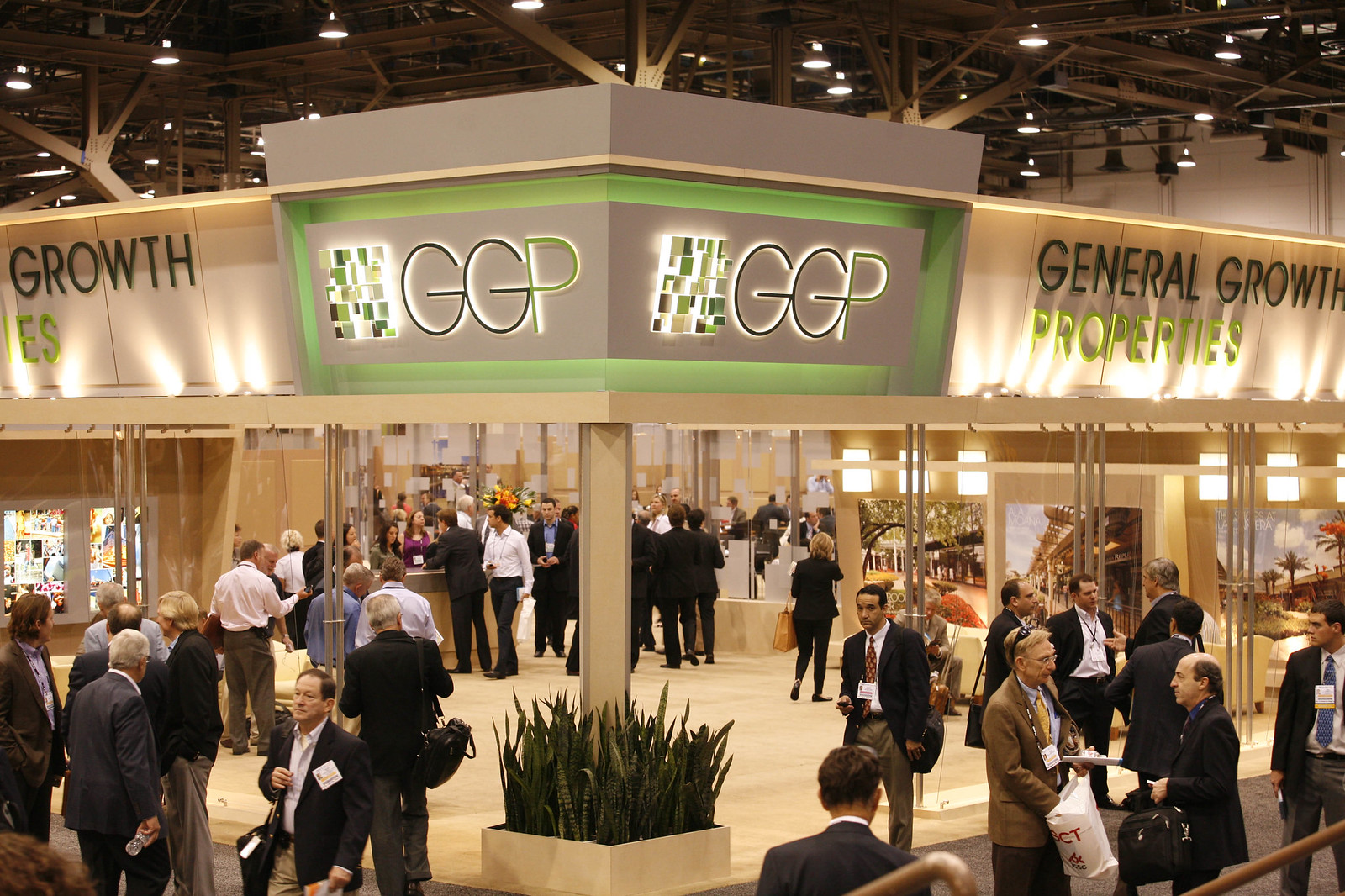This image depicts a bustling scene inside a large, modern convention center. Dominating the center of the space is an expansive and stylish booth belonging to "General Growth Properties" (GGP), with its name prominently displayed in black and green text. The ceiling above is an open concept with visible metal beams and lighting fixtures, giving the space a spacious and airy feel. The booth area resembles a mini mall, complete with various sections for attendees to explore.

A diverse crowd of professionally dressed individuals is present, many in black suits and ties, all carrying bags likely filled with promotional items or "schwag." They are mingling, talking, and examining the different exhibits available within the convention center. Some individuals have name tags and stickers on their jackets, indicating it's a formal event. Additionally, there are elements like aloe plants growing up the beams, adding a touch of nature to the otherwise sleek and modern setting. The overall atmosphere is lively and energetic, suggesting a professional gathering or celebration.